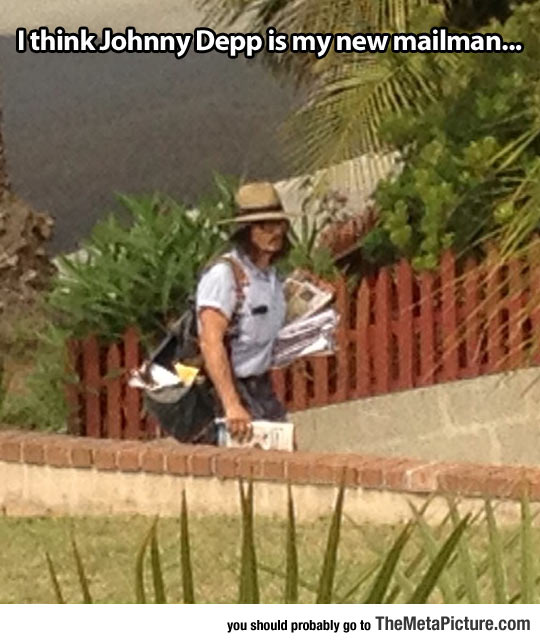The image is a humorous meme depicting a mail carrier who bears a strong resemblance to Johnny Depp. At the top of the meme, white text reads, "I think Johnny Depp is my new mailman." The mailman, a male with long hair, a mustache, glasses, and wearing a fedora, is dressed in a light blue shirt with gray work shorts. He is holding a mail bag and has a bundle of mail in his left hand while a magazine protrudes from his right hand. The scene appears to be taken from inside a residence, showing a walkway with a brick and cement wall on one side and a red wooden fence on the other. The front yard is grassy, with bushes and a hint of water or an ocean in the background. The primary colors in the image are tan, rust, green, and light blue. At the bottom of the meme, dark letters urge viewers to visit "themetapicture.com."